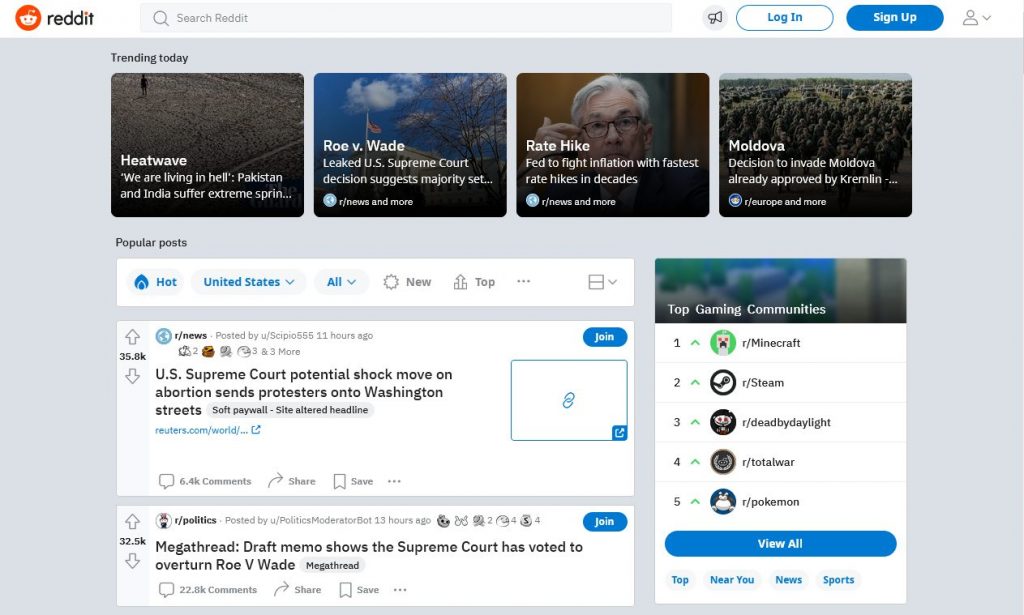The image depicts the homepage of Reddit with a light purple background and a white header at the very top. In the upper left corner, the black text "Reddit" is situated next to the recognizable Reddit logo featuring the iconic orange and white alien mascot. Adjacent to this is a light gray search bar with the placeholder text "search Reddit" and a magnifying glass icon. To the right of the search bar are buttons for "Log In" and "Sign Up." Further to the right is a user profile icon accompanied by a drop-down arrow.

Beneath the header, on the left side of the page, bold black text reads "Trending today." Below this heading are four rounded-corner squares arranged horizontally, each containing an image and a title in white text. These titles indicate the trending topics: "Heat wave," "Roe v. Wade," "Rate hike," and "Moldova," with each topic also featuring a brief description in thinner white text.

Further down the page, a section titled "Popular posts" is marked in bold black text. Within this section, a white stripe spans across the page, featuring filter options in bright blue text: "Hot," followed by location filters "United States" and "All." To the right of these options, filters "New" and "Top" are displayed in gray text.

The content beneath this filter section begins with a post from the subreddit r/news. The post is headlined "U.S. Supreme Court potential shock move on abortion sends protesters onto Washington streets," and has garnered 35.8 thousand upvotes and 6.4 thousand comments. Below this post, there is another article from the subreddit r/politics.